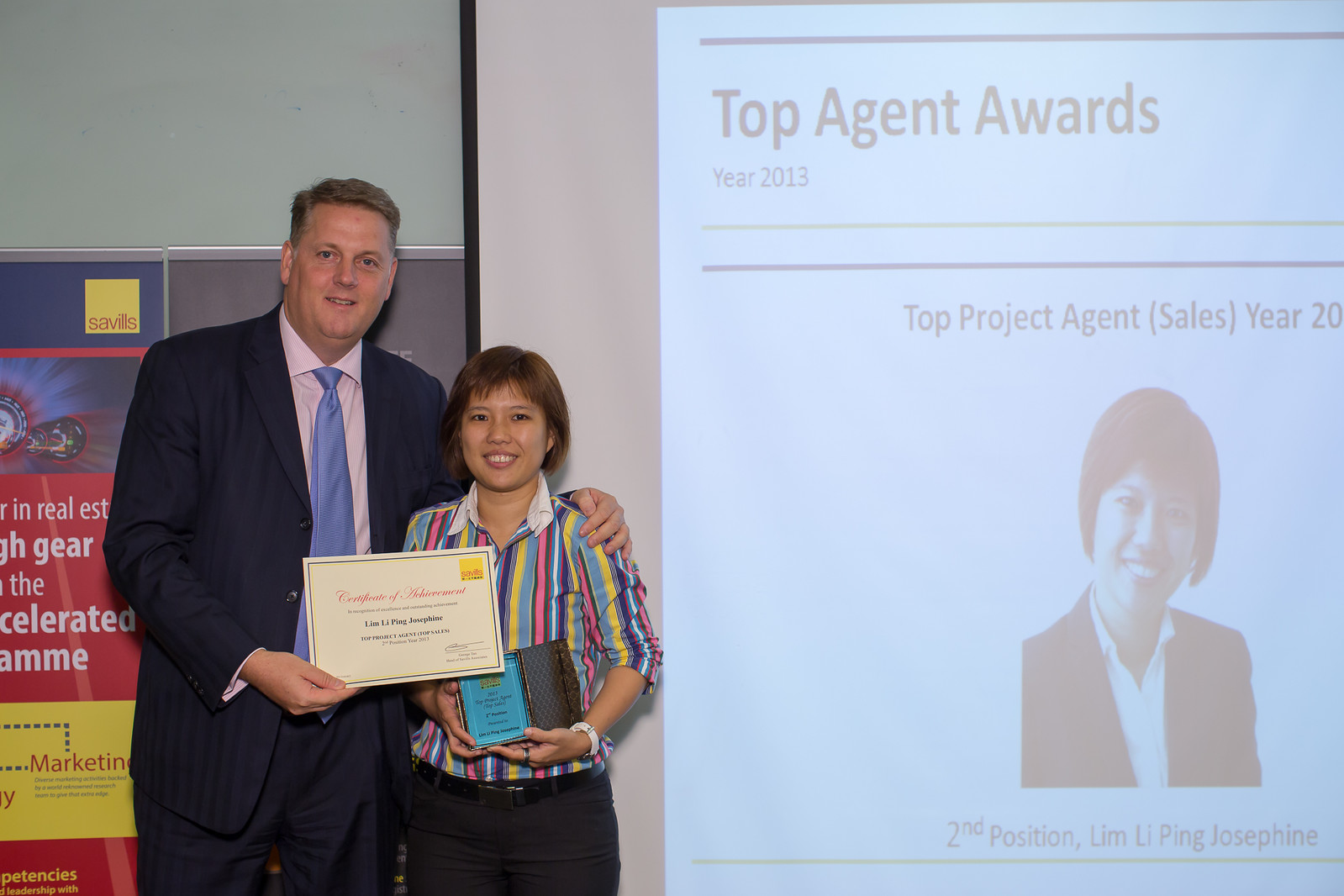The image depicts a poignant moment at an awards ceremony. Centered in front of a projector screen, a man in a black suit with a blue or purple tie stands beside an Asian woman, who has dark hair and olive skin. She's dressed in a multicolored, striped collared shirt and black pants. The man is handing her a certificate while she holds a plaque, indicating she's receiving an award. The projector screen behind them displays text in black writing that reads "Top Agent Awards." It shows a picture of the woman in a suit coat and white shirt with additional accolades such as "Top Project Agent Sales Year." The year mentioned, although partially cut off, references the year 2013. Behind them, vibrant red and yellow signs with the word "marketing" add a backdrop to the celebratory scene.